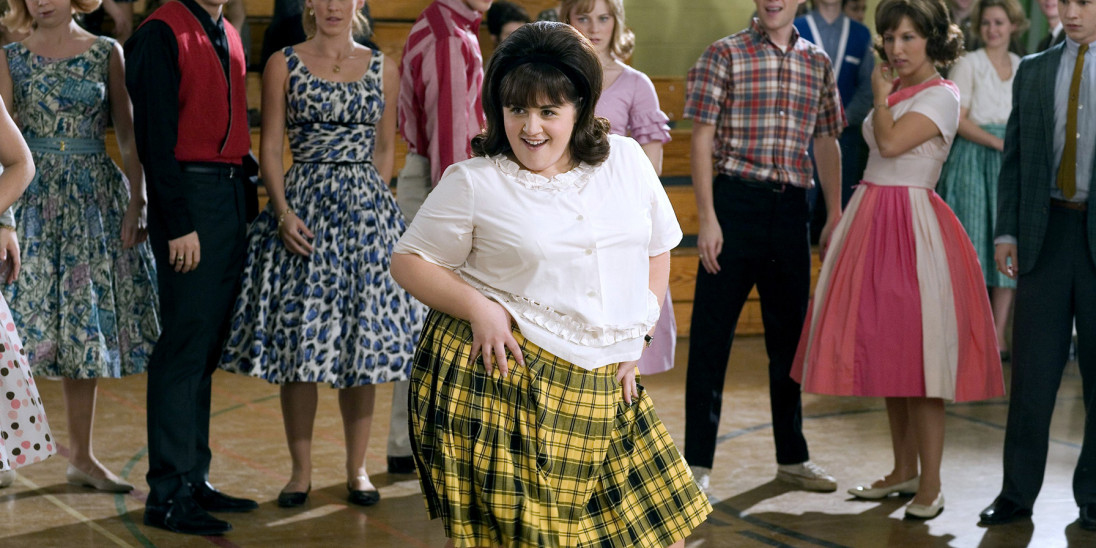This vibrant color still is from the movie Hairspray, likely the remake. At its center is an exuberant, plus-sized white woman commanding attention as she dances joyfully. Her hair, styled in an elaborate honey bee or beehive updo, is a dark brown shade with waves or curls ending above her shoulders. She is dressed in a white, short-sleeved button-up blouse featuring a ruffled collar and hem, paired with a knee-length yellow skirt adorned with green checkers in a pleated style. Her right arm is poised on her hip, accentuating her confident dance moves, and she's beaming with a smile. The scene unfolds in what appears to be a 1950s dance hall, possibly a gym, as indicated by the basketball court floor and bleachers in the background. Surrounding her are other elegantly dressed individuals in muted colors, with the men in suits and ties, some in red vests, and the women in classic dresses. The onlookers appear slightly bewildered, perhaps in disbelief at how well she dances despite her size.